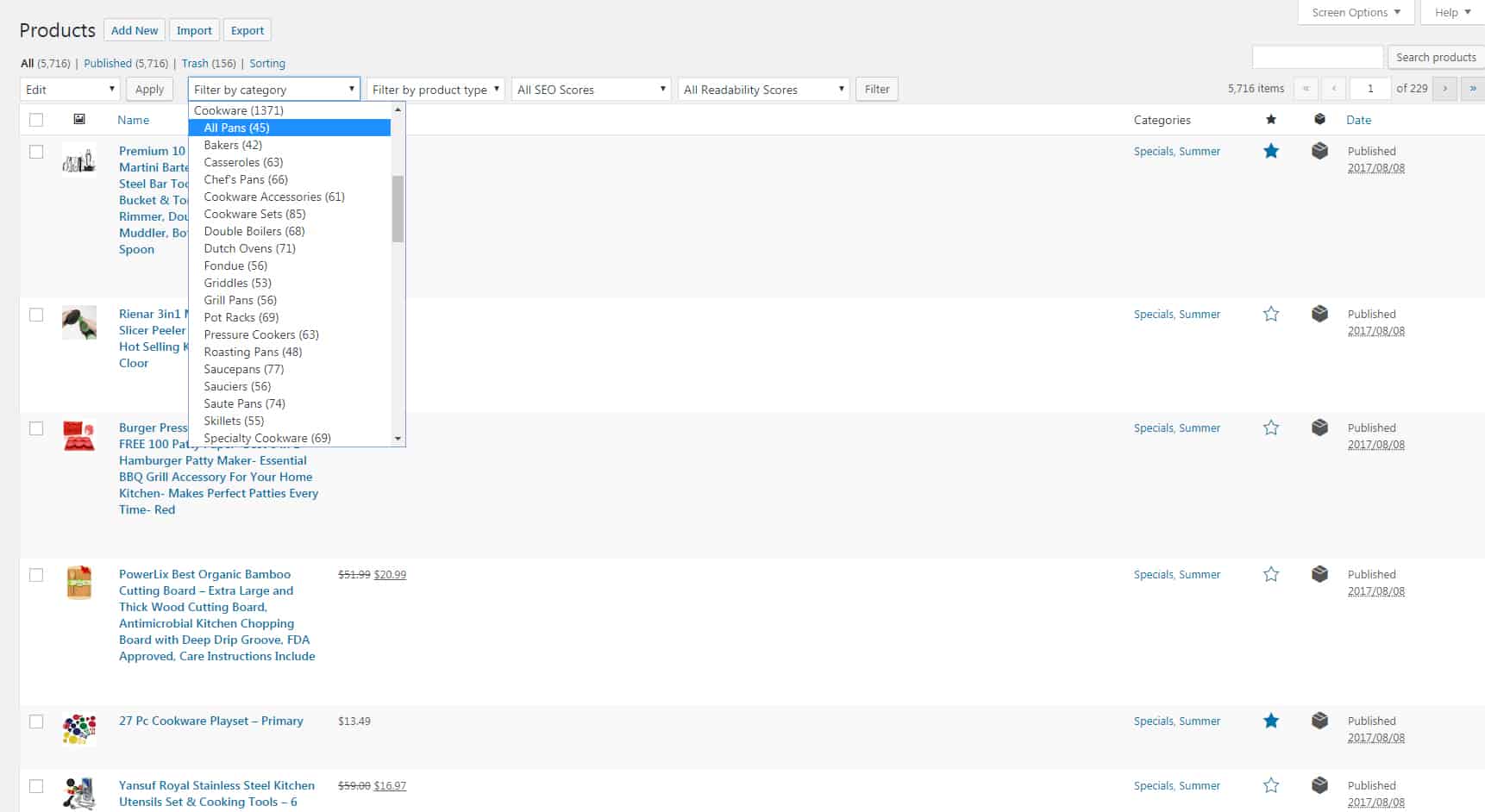The image showcases a captured menu or webpage from what appears to be an online shopping site. The design features a gray and white background with teal and gray text accents. At the top, there is a gray navigation bar with options such as "Products," "Add New," "Import," and "Export." The interface indicates that all products are published with additional functions for editing, applying changes, and filtering by category.

The filter categories listed include various kitchen-related items such as "Bakers," "Grit Pans," and "Fondue," among others. There is also an option to filter by product type and optimize SEO scenes. A search bar is present, allowing users to search through the products. It is indicated that there are 229 pages of results to browse.

As you scroll down, the page displays various items, including a bamboo item, a red item, and multiple pieces of cookware and utensils, totaling about six visible products. To the side, there is a categories section labeled "Summer Specials." Each item is accompanied by a series of teal-colored stars, gray boxes, a "Published on" date, and a square checkbox next to it.

Overall, the layout is designed for efficient product management and browsing within an online shopping environment, providing multiple filtering and sorting options to enhance the user experience.